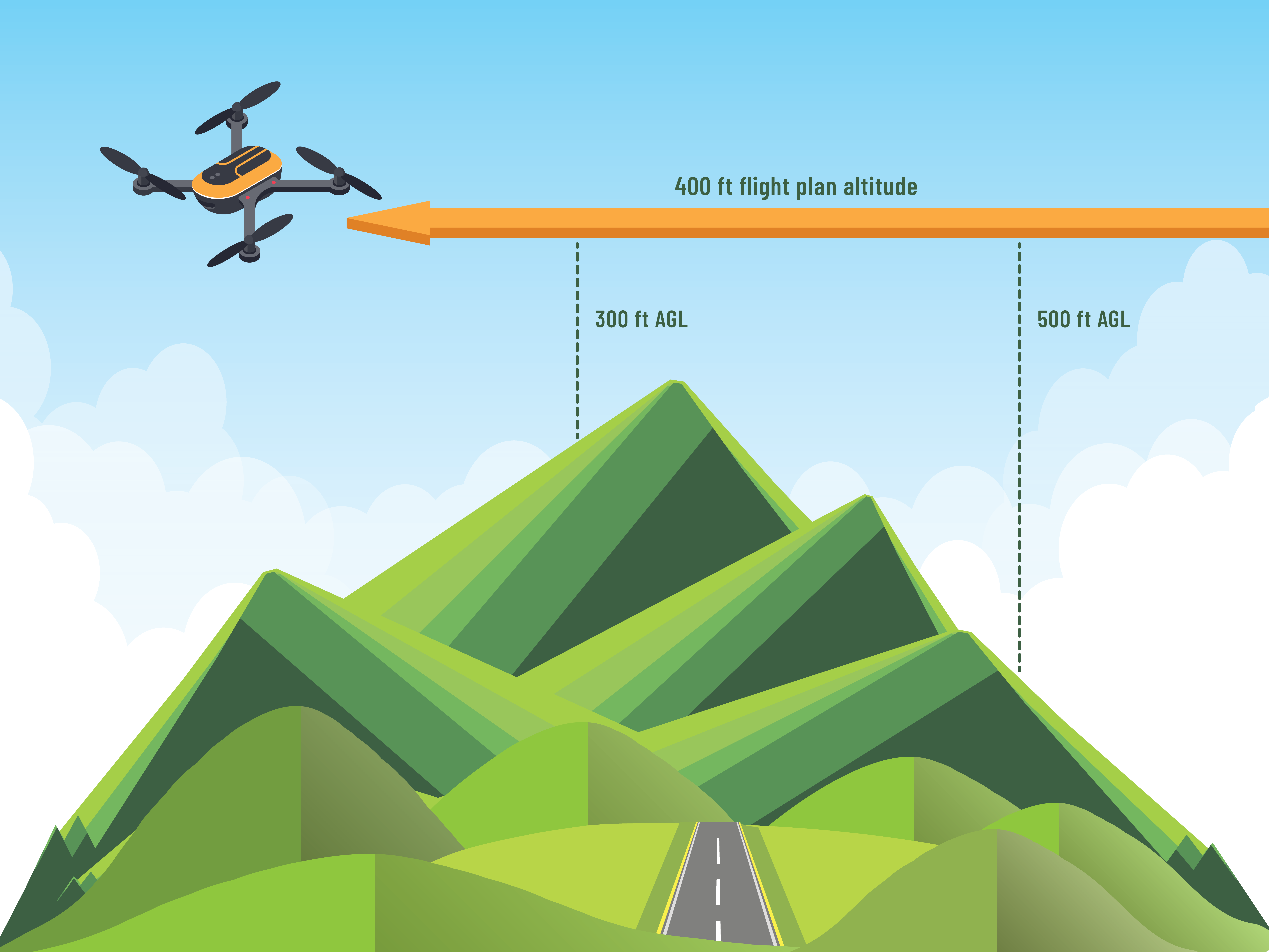The image is a detailed digital diagram showcasing a drone flight plan over a landscape. The scene features green hills presented in triangular shapes, each with dark green or almost black shaded areas on the right side. Central to the composition is a gray asphalt road marked by yellow borders and white dashed lines running down the middle. The sky is a light blue with fluffy white clouds dispersed on both sides. An orange and black drone with four propellers hovers on the left side of the sky. From the top right corner, an orange arrow points towards the drone, labeled in black with "400 feet flight plan altitude." Dotted lines extend from this arrow, meeting the hills and indicating altitudes of 300 feet AGL on the left and 500 feet AGL on the right. The overall format of the image is a landscape layout, emphasizing the expansive view of the terrain and the drone's altitude data.